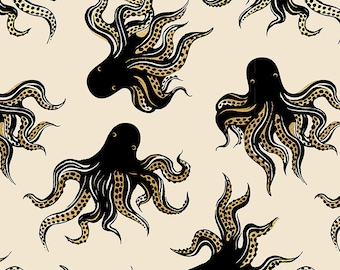The image is an old-timey drawing that resembles a wallpaper, featuring a repeating pattern of black octopi set against a beige cream background. The octopi are rendered from various angles, with distinct head tilts that add to the dynamic composition. Three full-bodied octopi are prominently visible, while parts of tentacles from additional octopi extend into the frame, enhancing the layered effect. Each octopus is adorned with dead yellow eyes, and the inside of their tentacles display a light orange hue with occasional white stripes and even black spots. The detailed tentacles contribute to the intricate pattern, which lacks any facial features but uses subtle moon shapes to suggest eyes. The quality of the image is fairly good, capturing the fine details and texture of the art.